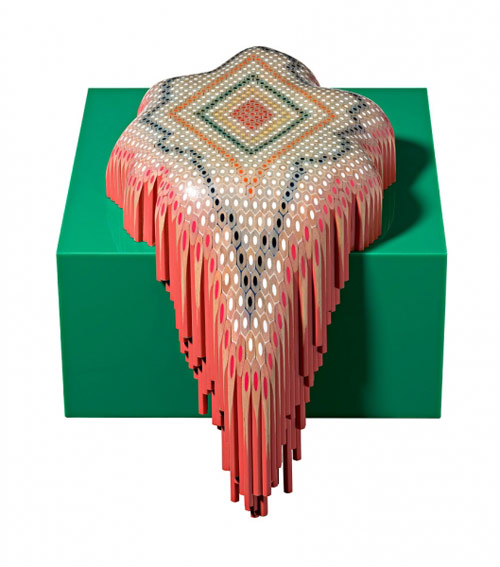The image features a smooth, teal-green cube serving as a base for a draped decorative fabric. The fabric, which appears to cloak an undefined object with irregular, bulbous edges beneath, showcases a vibrant, multi-colored tile pattern. Dominating the fabric's design is a central reddish-orange diamond. Surrounding this main diamond are progressively larger diamonds, incorporating various colors including yellow, teal, white, orange, dark blue, and black, all arranged in intricate, dot-lined borders. The fabric, possibly reminiscent of Native American or South/Central American designs, cascades over the front of the cube with an intriguing, fringed edge of pinkish hue.